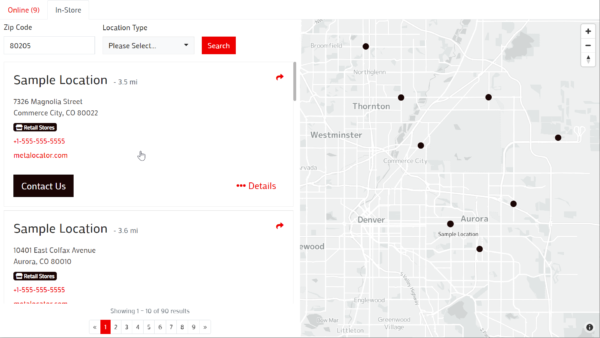The image depicts an online map application interface, devoid of any visible branding or markings. At the top of the interface, there are sections labeled 'Online,' 'In-Store,' and a ZIP code field displaying '80205.' There is also a drop-down menu under 'Location Type' and a prominent red search button.

The right side features a mostly desaturated map displaying various cities, including Denver, Arvada, Westminster, Thornton, and other surrounding areas. The map appears in shades of gray with subtle hints of pink and yellow.

Below the map, sample locations are listed. The first entry is 'Sample Location,' located 3.5 miles away at 7326 Magnolia Street, Commerce City, Colorado, 80022. The listing includes the label 'Retail Stores,' a placeholder phone number '15555555555,' the website 'metalocator.com' in very small text, a 'Contact Us' link, and a 'Details' option in red.

The second sample location is 3.6 miles away at 10401 East Colfax Avenue, Aurora, Colorado, 80010, with identical placeholder phone information and similar additional links.

At the bottom of the interface, navigation elements show '1 - 10 of 90 results.' An interactive pagination system allows for scrolling through search results with backward and forward arrows. The number '1' is highlighted in a red square, indicating the current page.